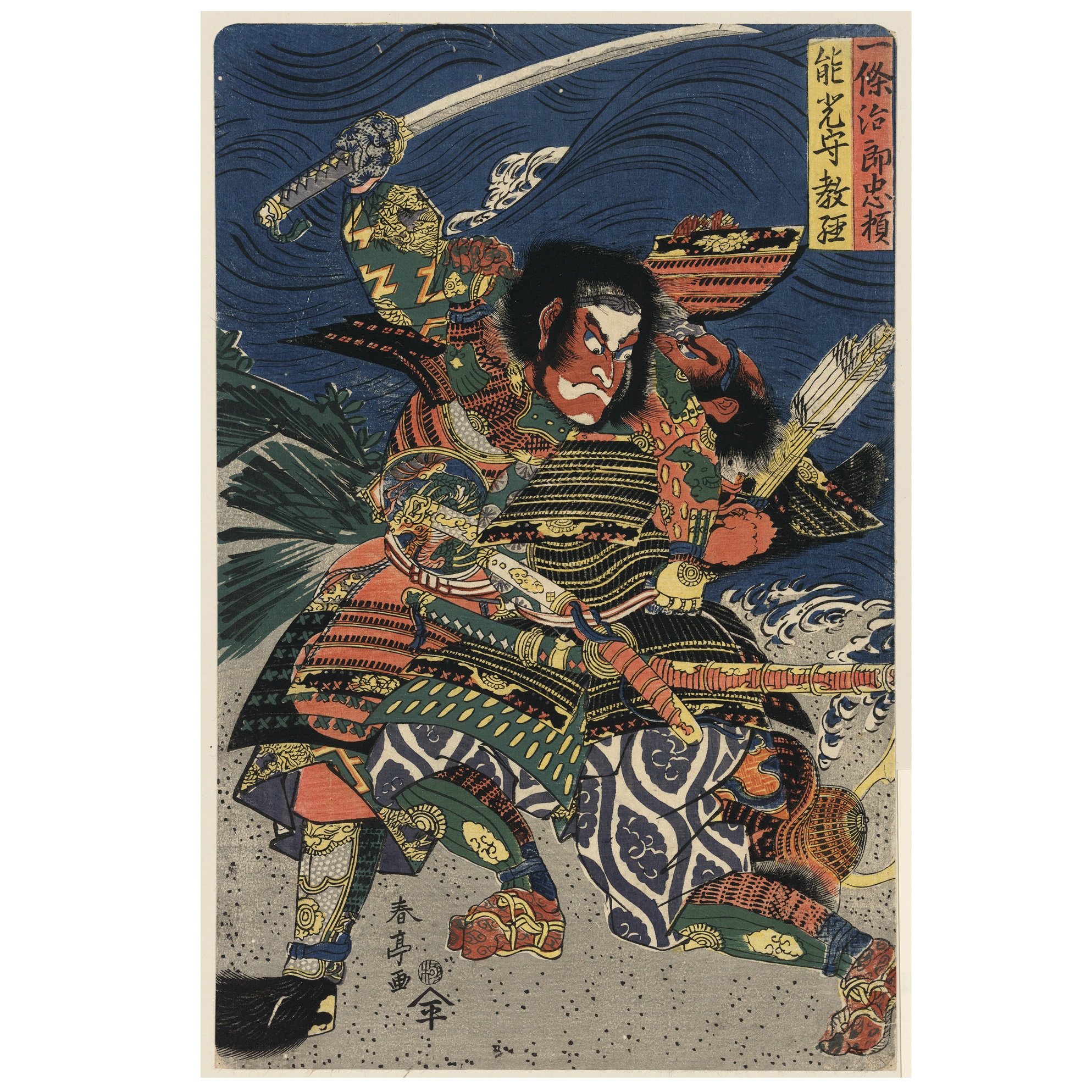The photograph captures the front of a card featuring an intricately hand-drawn image of an Asian warrior. This warrior is depicted with dark hair and a distinct brownish-red face. He wields a sword high above his head, suggesting a dynamic pose. His attire is remarkably colorful, with fabrics displaying a mix of blue, white, yellow, green, and the same brownish-red hues. Patterns and accents of black and green further embellish his clothing. The scene reveals that the warrior is engaged in combat, as evidenced by the presence of another figure whose face is partially visible, hinting at a confrontation. At the top right corner of the card, two vertical triangular strips in yellow and brownish-red feature Asian script, adding an authentic cultural touch. The background consists of a stark black section transitioning into a gray surface upon which the figures are positioned, providing depth and contrast to the vivid characters.